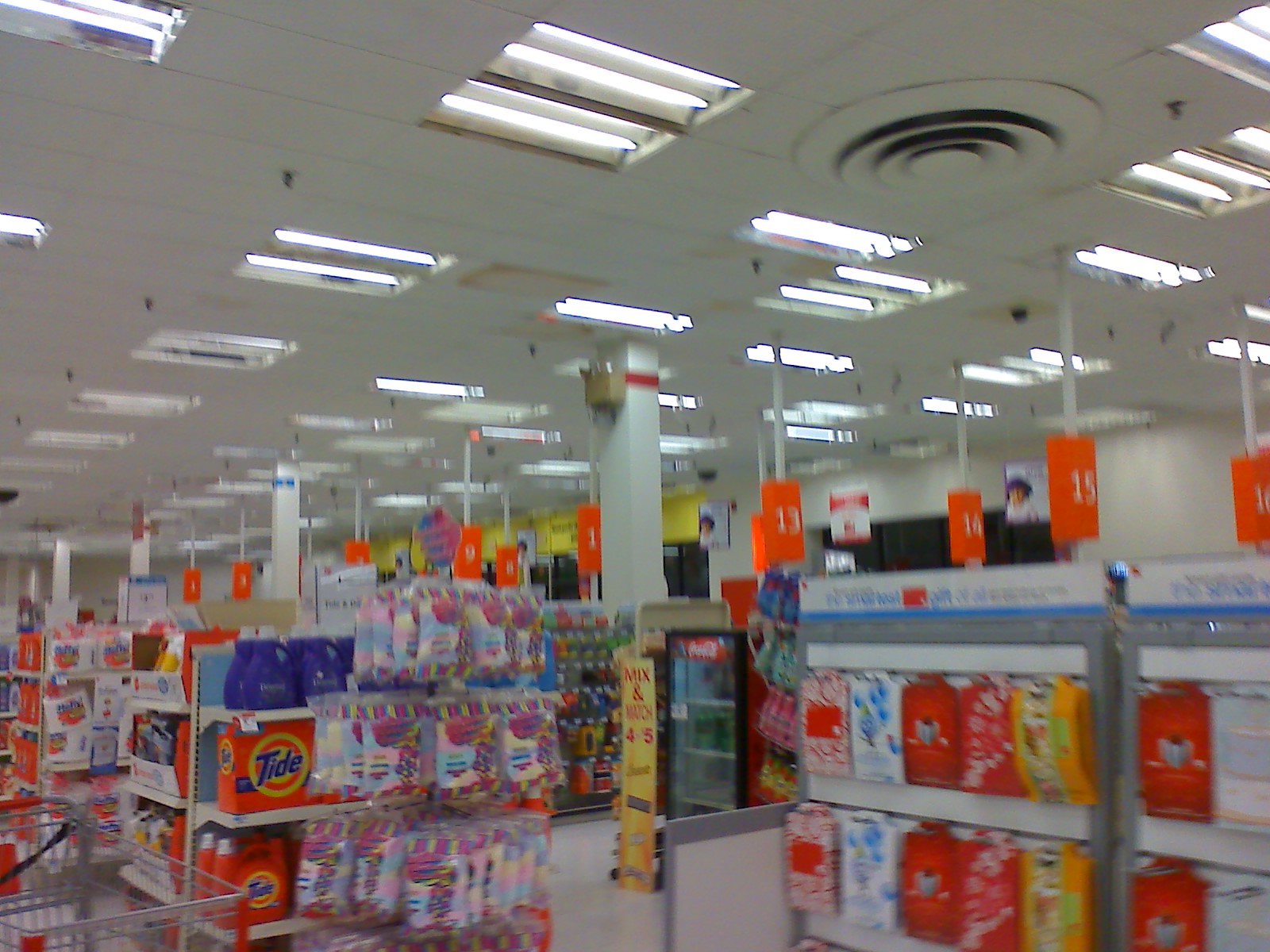The photograph depicts a blurry, out-of-focus scene inside a large box store, possibly a department or grocery store. The white ceiling is dominated by rows of recessed troffer fluorescent lights, each housing two or four tubes, along with large circular air vents and sprinkler heads. The scene includes multiple aisles, identifiable by round or square posts, each marked by bright orange signs with white numbers that are easy to read. These signs indicate aisle numbers 13 through 16, progressing towards the back of the store.

In the lower right corner, there are racks, possibly holding cough drops or gift bags, though the details are unclear due to the photo's blurriness. A central display prominently features various Tide laundry detergents: powdered Tide in boxes on the middle shelf and large jugs of liquid Tide on the bottom shelf, alongside other blue bottles that might be Downy fabric softener or another type of liquid detergent.

On the left side of the image, there's a hint of checkout lanes, or perhaps another aisle, and what looks like a refrigerated case potentially holding drinks. Additional details include a yellow sign with a mix-and-match offer for $5, featuring images of candy bars beneath it. In summary, despite the lack of focus, the image captures a bustling store environment characterized by structured aisle markings and a variety of brightly colored products on shelves.